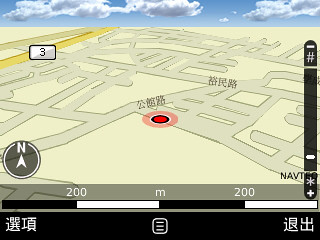This image appears to be a screenshot taken from an older model Garmin GPS system. The display prominently features Chinese characters, indicating that the location is somewhere in China. A compass is situated in the bottom left corner, accurately pointing north. The bottom corners of the image also contain additional Chinese text. The individual's current position is marked with a distinct red circle dot. Several streets labeled in Chinese are visible, providing a context of urban navigation. The upper portion of the image showcases a sky filled with a scattering of clouds against a blue backdrop. The GPS interface itself has a yellowish hue, reflecting the design aesthetics of older GPS technology.